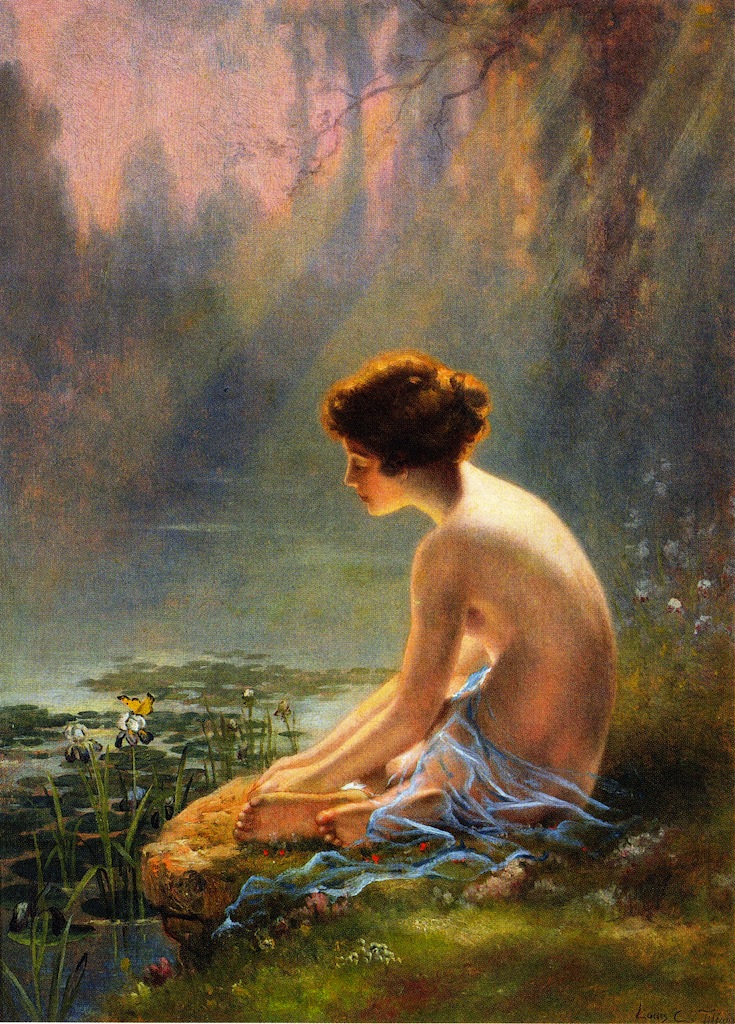This image, titled "Seated Nude at Lily Pond," is a color painting by Louis Comfort Tiffany, created in the early 1900s in the Art Nouveau style. It depicts a young, mostly nude woman with dark reddish-brown hair, styled in a 1920s fashion, seated on grass by the side of a pond. Her feet dangle in the water. She is draped in a light blue, sheer gossamer cloth that covers her lap and genital area, appearing almost illuminated and otherworldly.

The scene is outdoors, with the woman positioned cross-legged or with her knees to the side, looking downward at two ducks and floating lily pads in the pond. The water is adorned with green vegetation and yellow and white lilies. Her posture has her elbows resting on her legs, bent slightly towards the water, which enhances her peaceful demeanor.

Surrounding her is a richly detailed setting: a forest in the background, depicted with a pointillism-like texture that feels dotted and impressionistic. The trees are light green, casting long, thick beams of sunlight that stream through the branches and create a luminous orange-pinkish glow, particularly illuminating her back. The background remains blurry, emphasizing the serene and ethereal quality of the entire composition.